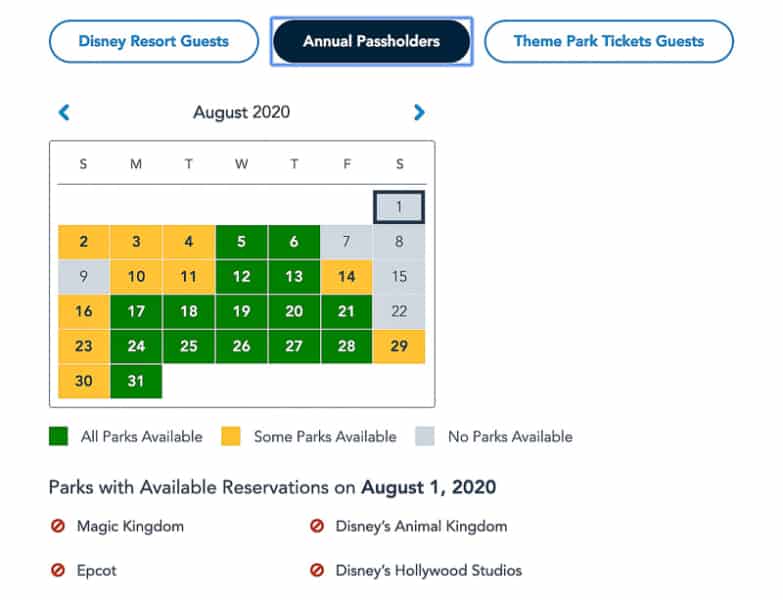The image is a detailed screen capture of a calendar for August 2020, specifically for Annual Pass Holders of Disney Resorts. The calendar is color-coded to indicate park availability for each day. At the top of the screen, categories such as Disney Resort Guests, Annual Pass Holders, and Theme Park Ticket Guests are listed, with the Annual Pass Holders tab currently selected.

The key below the calendar explains the color codes: 
- Green indicates "All parks available",
- Gray signifies "No parks available",
- Yellow shows "Some parks available."

For August 1st, 2020, a Saturday, the calendar displays gray, signifying no available park reservations. Additionally, a note at the bottom lists the availability of specific parks for that day: 
- Magic Kingdom: No,
- Epcot: No,
- Disney's Animal Kingdom: No,
- Disney's Hollywood Studios: No. 

The capture implies that most Saturdays in August are fully booked, reflecting the high demand and limited availability during this period.